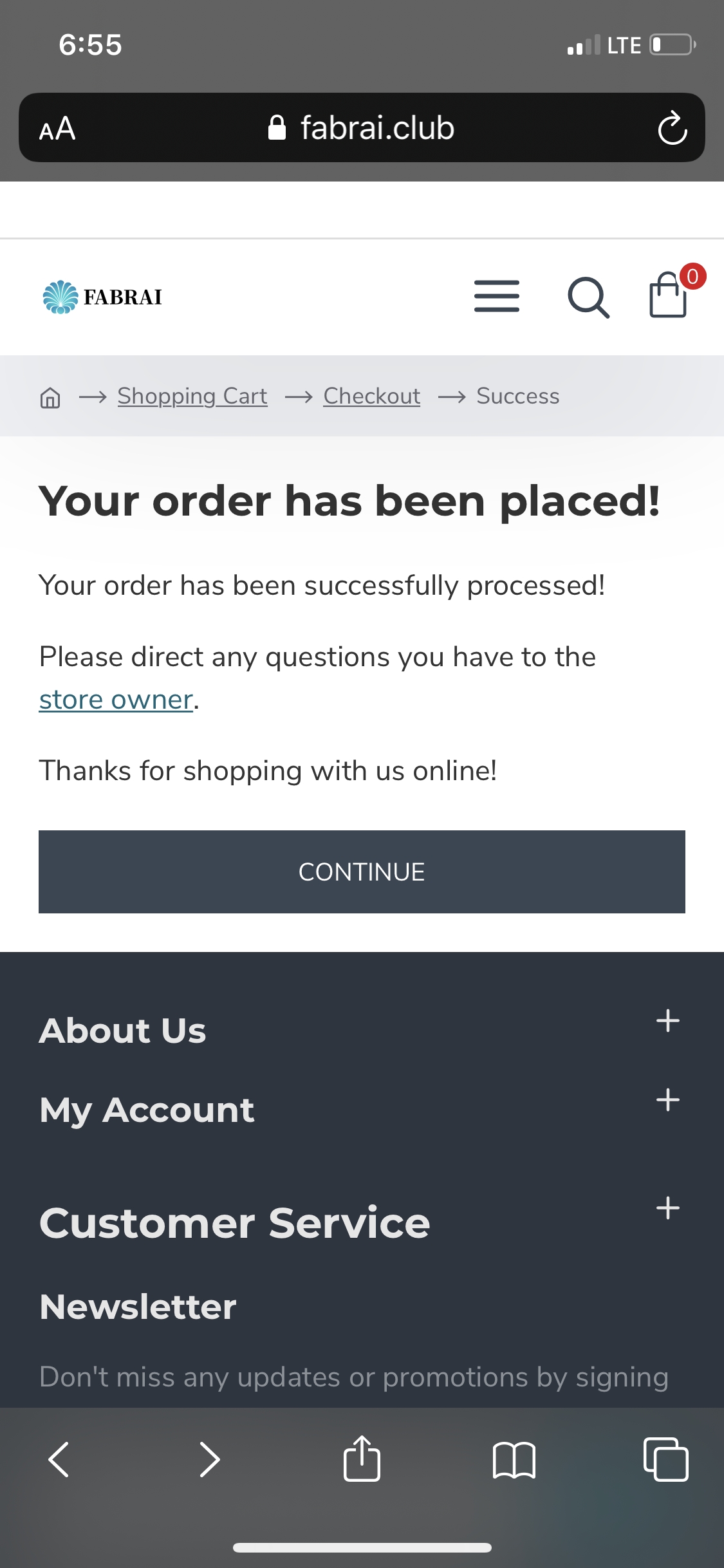In the midst of a tense forest clearing at dusk, a group of survivors are on high alert, frantically preparing for an imminent attack. A sense of urgency permeates the camp as one of the leaders urgently exclaims, "I'll get you the supplies. But there's no cure. The grounders don’t use the sickness to kill." Another, more skeptical voice retorts, "Really? Tell that to them."

Tensions rise as the group reacts to the news, "I warned you about seeing that grounder again," one of the survivors admonishes. Defiantly, another responds, "Yeah, well, I have a warning for you too. The grounders are coming and they're attacking at first light." Amid the frantic preparations, someone shouts, "Come on, help me get Clark into the dropship!"

Questions about their defenses arise, "How many bullets can you make by first light?" someone inquires anxiously. A grim reply follows, "I don't know, it'll take me years to get talking to them. It'll get better. If he's not sick by now, then he's probably immune, like me." As they move to usher Clark to safety, one of them assures, "Yeah, come on, she can take one."

In an effort to strategize, another asks, "What else did Lincoln tell you?" The reply offers a glimmer of hope, "The virus doesn’t last long. I feel better. They need to stay hydrated. You need to stay hydrated." In the last moments of daylight, orders are given, "Okay, send two," as the group steels themselves for the impending attack.